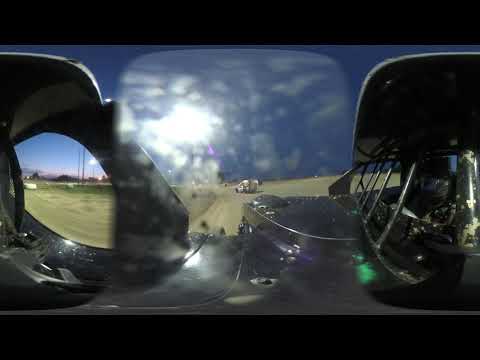The photograph, appearing to be taken from within a vehicle, is highly distorted and blurry, possibly taken with a webcam or using panorama technique. The main focus is through a windshield, revealing a dirt racetrack stretching into the background and curving off to the left, under a blue sky with sunlight causing significant glare. Directly ahead in the distance, a white vehicle, likely a van or race car, is visible, showing its side profile with the hood facing left. The foreground of the image is dominated by black interior elements and instruments of the vehicle, and the right and left edges of the image appear bubbled and pixelated, suggesting multiple views stitched together. The right side shows a black helmet with a screened face area, possibly the driver, adding to the impression of a racetrack scene, while the left side hints at more of the track or possibly a pit stop area. A tall light can be seen far off in the distance as the sky begins to darken.